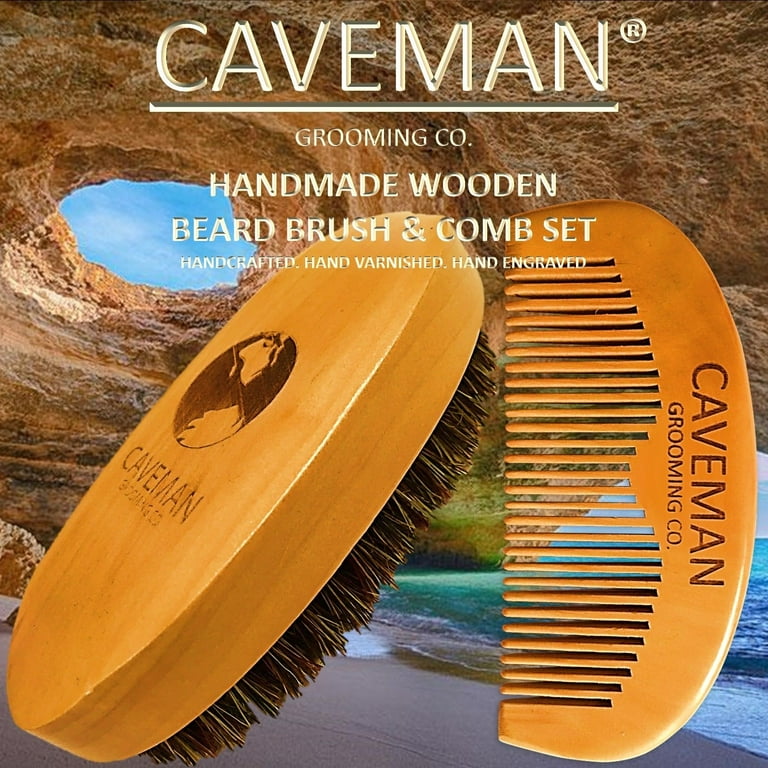This advertisement for the Caveman Grooming Co. features a meticulously illustrated handheld beard brush and a curved comb, both crafted from light wood. At the top of the poster, the brand name "Caveman Grooming Co." is prominently displayed in bold white letters. Below, it highlights the handmade nature of the wooden beard brush and comb set, emphasizing that each piece is handcrafted, hand varnished, and hand engraved. 

The brush itself is presented with light wood and brown bristles, featuring a distinctive emblem on the back that resembles a globe split into dark brown and gold, with the brand name centered. To the right of the brush, the comb is depicted with black lettering stating "CAVEMAN GROOMING CO."

The backdrop of the advertisement includes a serene beach scene, with a striking rock formation jutting out over sandy shores and blue-green ocean waters, hinting at a natural, rugged aesthetic that complements the brand's "Caveman" identity. The visual theme encapsulates earthy tones of light and dark brown, punctuated by crisp white text and the soothing hues of the seascape, creating a harmonious and inviting appeal.